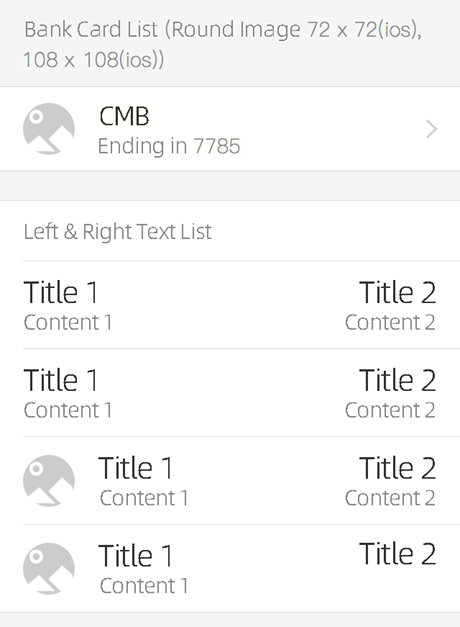### Detailed Caption for User Interface Design of a Financial Services Application

This image showcases a user interface design for a financial services or account management application. The primary focus is a bank card list section. It features a placeholder icon for a bank card that is displayed at multiple resolutions: 72 by 72 pixels and 108 by 108 pixels, optimized for iOS. 

Centrally displayed, the bank card icon comes with specific details such as the bank name "CMB" and a card number ending in 7785. Accompanying the bank card icon is a navigation arrow indicating that this item is interactive, allowing users to click for more details and actions.

The interface also includes a structured list of items presented in a left and right text format. Each item in this list contains:
- Main headings titled "Title One" and "Title Two"
- Subheadings labeled "Content One" and "Content Two" which provide additional details under each main heading.

The repetition of similar items within this structured list suggests that it could be used to display transaction records, notifications, or other categorized financial data. The meticulous layout of this section emphasizes delivering essential financial information clearly and organized, enhancing the user's ability to manage their accounts effectively.

The design likely serves to display linked bank cards, offering a brief overview with an option to delve into more in-depth information. The overall aesthetic combines functionality with a straightforward, user-friendly presentation tailored for financial and account management.